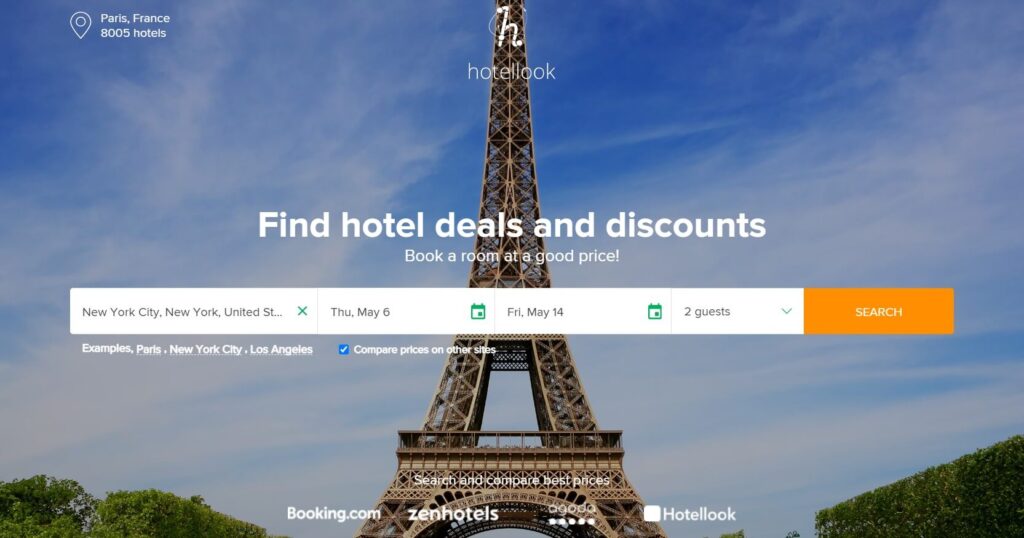This screenshot depicts a tourism booking website centered on a full-screen background photo of the iconic Eiffel Tower in Paris, France, against a vivid blue sky. The foliage and greenery frame the Eiffel Tower on either side, enhancing the scenic beauty. In the top left corner, a GPS icon accompanies a description indicating "Paris, France," followed by the number of available hotels: "8005 hotels."

The website belongs to a company named "Hotel Look," whose logo, featuring a prominent "H," is centrally placed. Below the logo, a bold heading declares, "Find hotel deals and discounts - Book a room at a good price!" Beneath this heading lies a search bar, pre-filled with an example search query that reads, "New York City, New York, United States Thursday May 6th to Friday May 14th, 2 guests." Next to the search bar, a vibrant orange button labeled "Search" encourages user interaction.

Additionally, the site offers an option to "Compare prices on other sites," supported by a secondary prompt to search and compare the best places on popular booking platforms such as Booking.com and others. The overlay, slightly darkened for readability, brings the various interactive elements into sharp focus, ensuring a user-friendly experience.